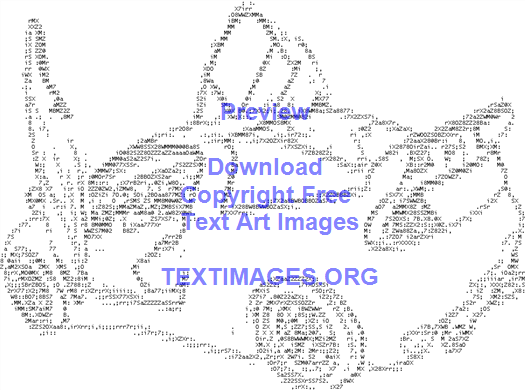In the center of this image is blue text that reads, “Preview, Download, Copyright Free, TextArt Images, TextImages.org.” Behind the text, there's a detailed drawing of a sporty car, depicted in a dot print manner reminiscent of ASCII art, where characters and numbers form the image. This car features doors that open vertically, resembling sliding wings, and lacks back doors, suggesting it only has seats for the driver and passenger. The car's profile is facing left, allowing a view of its side and a bit of its rear, where a prominent spoiler or fin is visible. You can make out some interior details including one of the seats and what appear to be gauges. The black and gray outline of the car evokes the look of an old 1995 printer output, complete with visible wheels and plated hubcaps. The entire image maintains a monochromatic, uncolored design, reinforcing its vintage blueprint aesthetic.